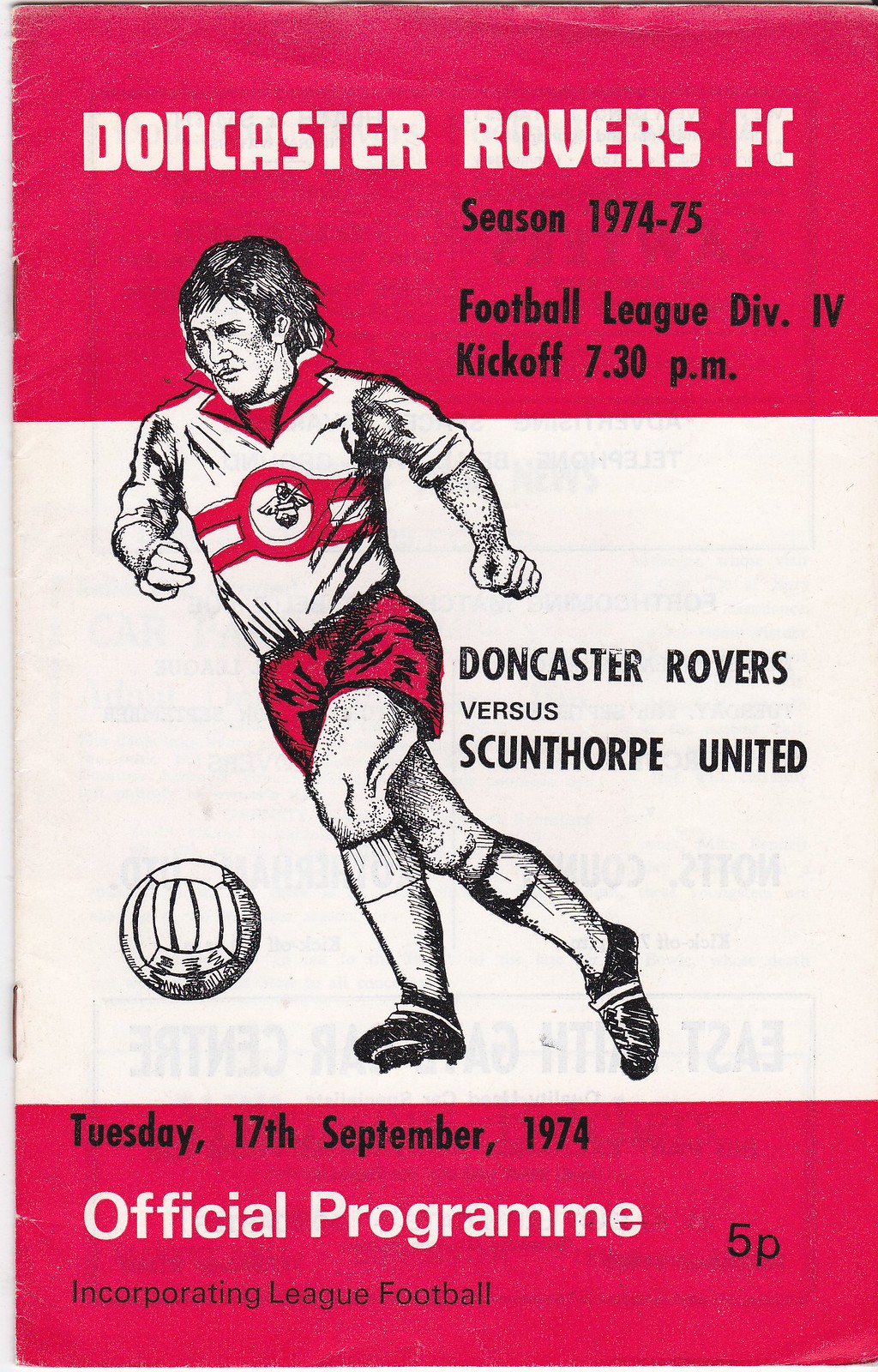This vertically aligned, worn booklet appears to be an official program from the 1974-75 season for a soccer match between Doncaster Rovers FC and Scunthorpe United. The background of the image is divided into three distinct color sections: the top is dark red, the middle is white, and the bottom is a very dark pink. The booklet is held together by two staples and shows slight wear and tear along the spine. At the top, in all caps white block letters against the dark red background, it reads "Doncaster Rovers FC." Below this, in black text, it states "Season 1974-75, Football League Division IV, Kickoff 7.30 p.m." Prominently displayed in the middle section against the white background are the words "Doncaster Rovers vs. Scunthorpe United" in black text. To the left, there's an outlined image of a soccer player wearing black shoes, red shorts, and a white and red shirt, with the soccer ball in mid-air. At the bottom of the page in the dark pink section, "Tuesday, 17th September 1974" is printed in black text. Beneath that, in white text, it says "Official Program," followed by "Incorporating League Football" in black text. To the right of this, also in black, the price "5P" is displayed.